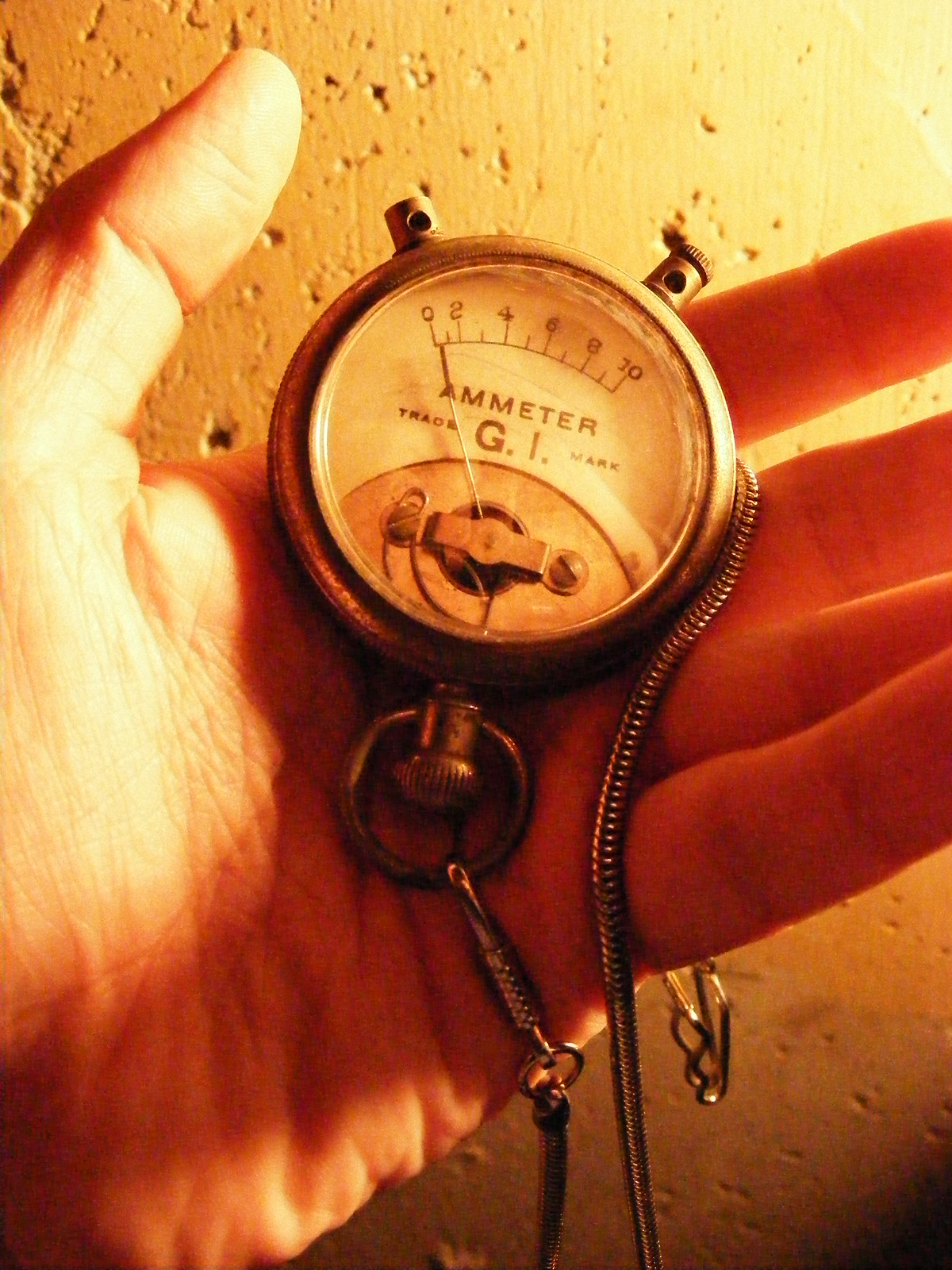This indoor photograph captures a detailed image of a Caucasian male's left hand, prominently displaying an ammeter device. The ammeter, resembling a round stopwatch, is light brown or possibly a bronze or silver color, with a complex surface texture. It is marked with the words "AMMETER" and "TRADE G.I. MARK," indicating its authenticity. The device features a dial ranging from 0 to 10, marked with additional shorter lines for finer measurements. Two cylindrical protrusions, including a knurled knob, are positioned at the top, suggesting buttons or connectors. A chain or coiled cord extends from the device, looping back behind it. The background reveals a stone or cork-like wall, pitted with porous holes and casting an orange hue, indicating dim or natural sunlight lighting. The man’s thumb is raised, highlighting his grasp on the ammeter and adding context to the scene.